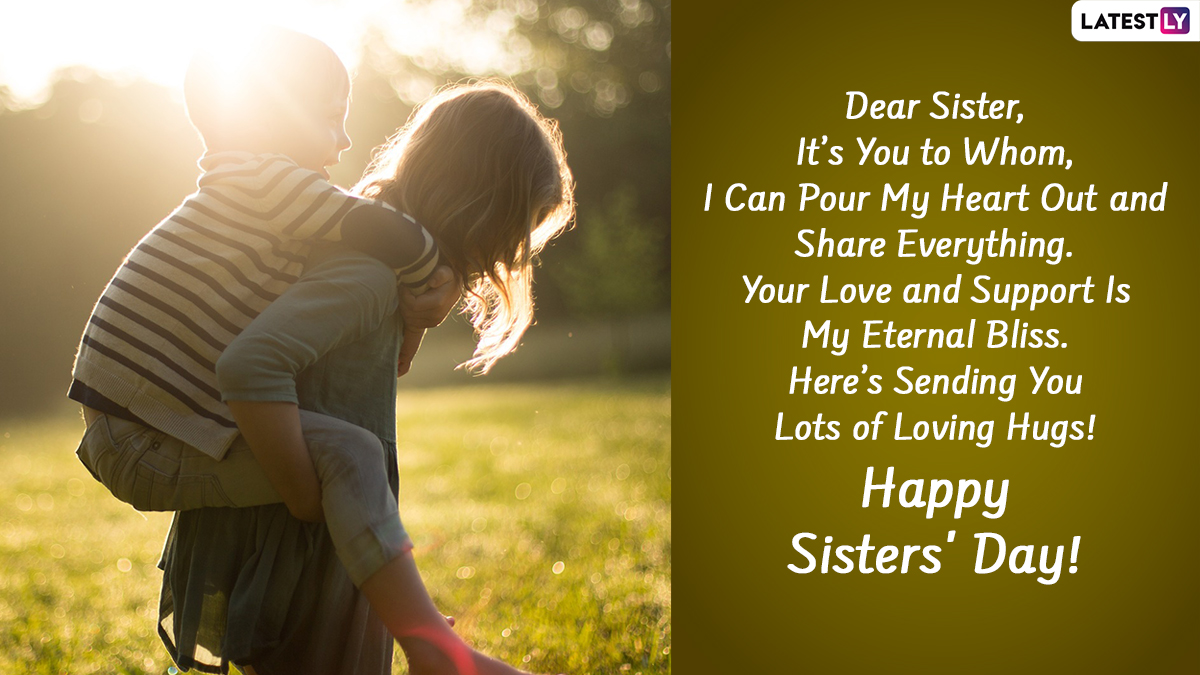The image is a beautifully crafted Happy Sister's Day card divided into two sections. On the left side, there are two children playing joyfully in a garden at sunset, their playful shadows cast by the golden light. The older child, a girl in a blue dress, is giving a piggyback ride to her younger brother, who wears a white and blue long-sleeved shirt paired with cropped jeans and bare feet. Her blonde hair partially covers her face, while he clings happily to her, his arms wrapped tightly around her neck. The background is softly blurred, highlighting lush vegetation that encircles the scene. On the right side of the card, set against an olive green background, is a heartfelt message written in white ink: "Dear Sister, it's you to whom I can pour my heart out and share everything. Your love and support is my eternal bliss. Here's sending you lots of loving hugs. Happy Sister's Day." The upper right corner features the brand logo of Latestly, with "Latest" in black block letters and "LY" in white block letters on a pink and purple gradient square. The entire composition exudes warmth, love, and the special bond shared between siblings.